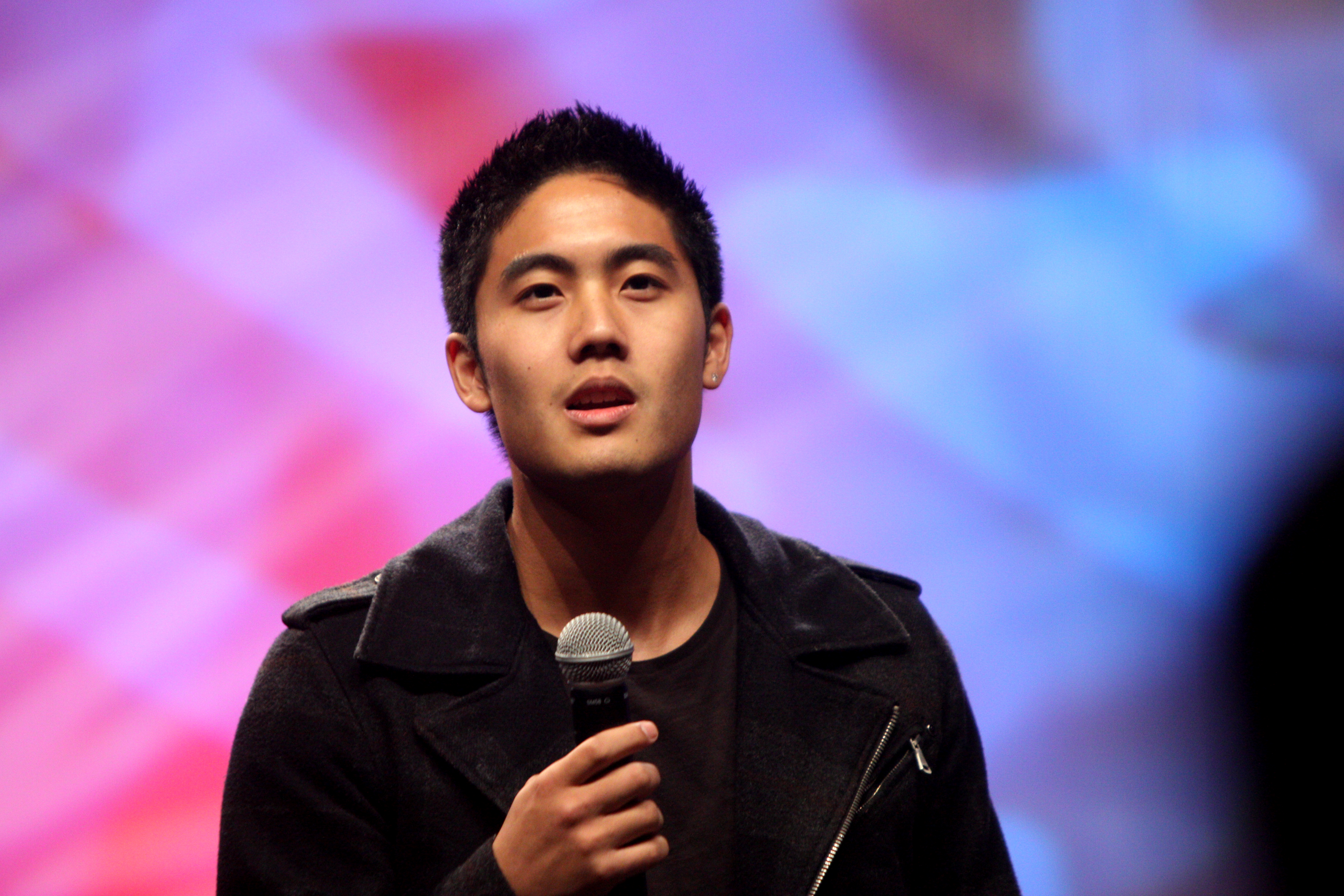The image depicts a young Asian man, likely in his mid to late 20s, standing on what appears to be a stage. He has short, spiky black hair, dark eyes, and a clean-shaven face. His mouth is open, suggesting he might be singing or speaking. He is wearing a black t-shirt underneath a fashionable black jacket with a silver zipper, which is unzipped. In his right hand, he holds a microphone, positioned in front of him. He is looking slightly upward, past the viewer, at something off-frame. The background is a blurry array of vibrant colors, including shades of blue, pink, purple, red, and black, possibly created by stage lights. The overall ambiance hints at a performance setting, enhanced by the colorful, checkered pattern of lights.